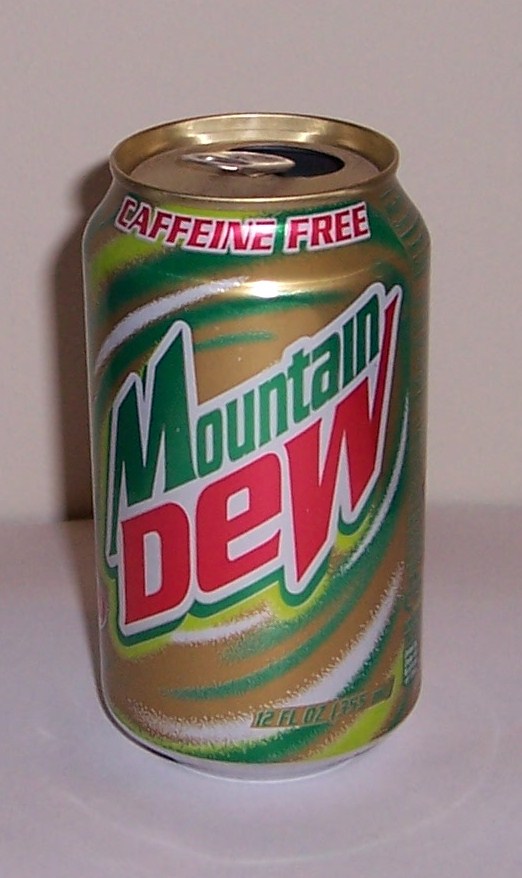A vertically oriented color photograph captures a can of Mountain Dew positioned centrally. The image is tinged with a magenta hue due to the lighting. The can features the iconic "Mountain Dew" branding in diagonal green, red, and white text ascending from the left to the right. Encasing the brand name is a vibrant, swirling pattern in shades of white, gold, green, and light green. At the top of the can, in bold red block letters outlined in white, the words "Caffeine Free" are prominently displayed. The can's top has a distinctive gold appearance. It rests on a table, and a subtle light reflection encircles the bottom of the can, adding a hint of luminosity to the background.